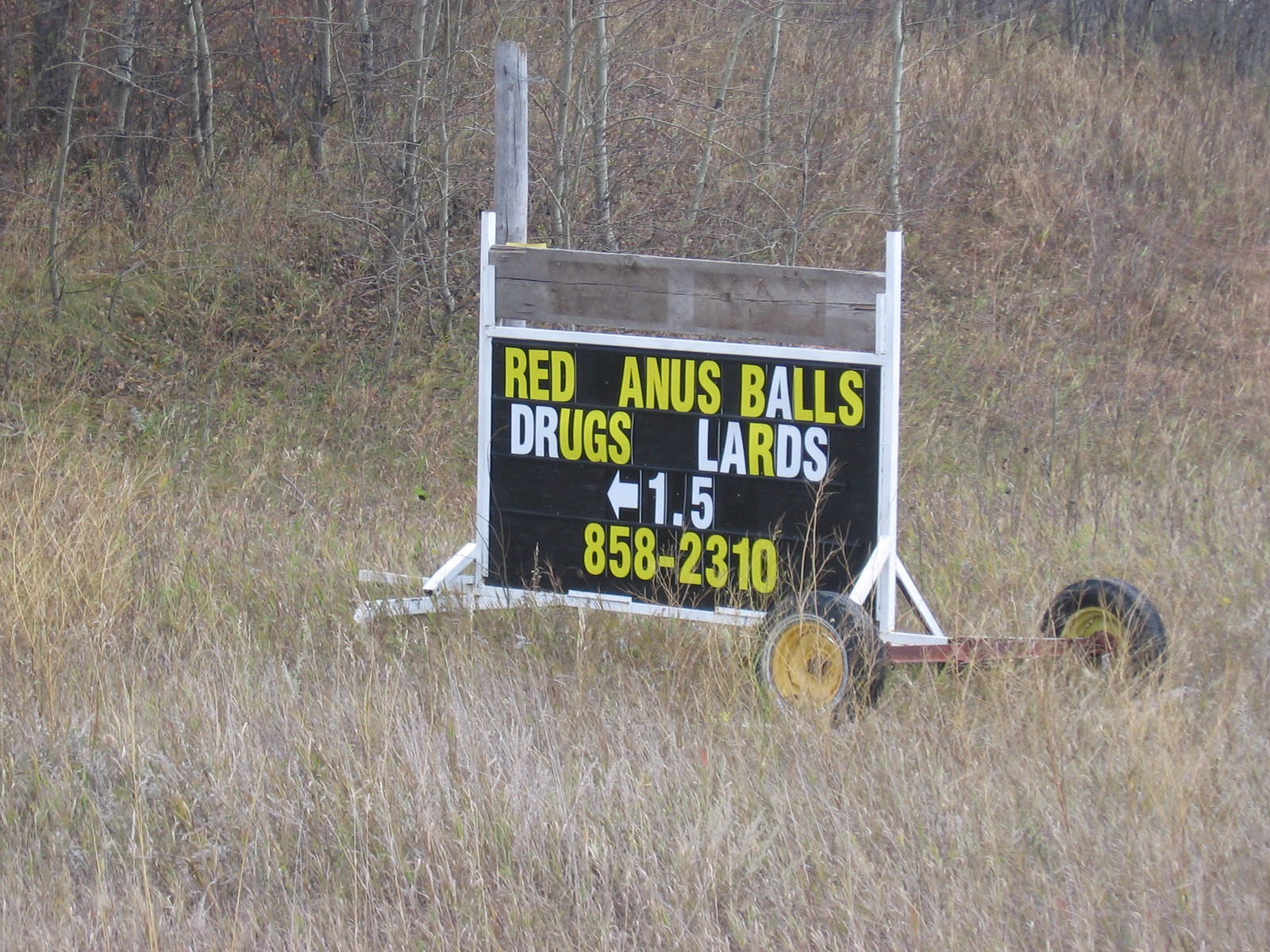The image captures an exterior scene with moderate lighting and a background of high, dried grass interspersed with the bases of gray-colored saplings. At the center of the frame sits a large, mobile billboard sign on a trailer rig equipped with wheels, black with yellow insides and a purple frame, allowing it to be pulled and moved. The sign itself, framed in white metal, is prominently set against a black background and features a wooden plank at its top. The text on the sign is arranged in a mix of yellow and white, reading "Red Anus Balls Drugs Lards." "Red" and "Anus" are yellow, while "Balls" is yellow except for the letter "A." "Drugs" features "DR" in white and "UGS" in yellow, and "Lards" is white except for the letter "R." Below this, an arrow points leftward alongside the text "1.5" in white. The bottom line displays a phone number, "858-2310," in yellow text.